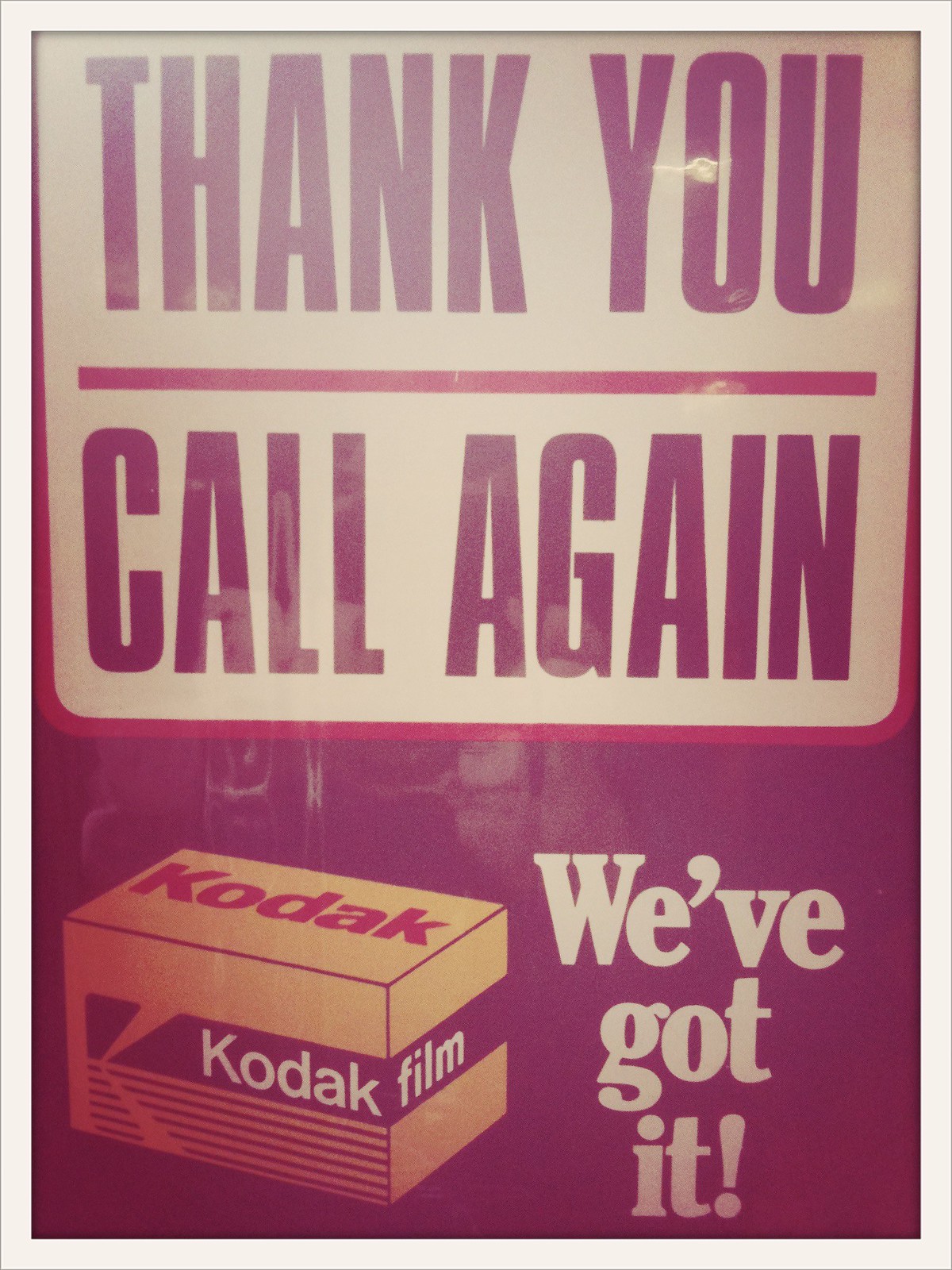The image showcases a vintage advertisement with a distinctly faded and dull aesthetic, reminiscent of the 1950s or 1960s, as seen through a glass window, suggesting an old storefront sign. The background is primarily purple, adding to the nostalgic vibe. Dominating the top portion of the ad is the message "THANK YOU CALL AGAIN" in black, all capital letters, separated by a red line. Below this sign, there is a depiction of a small, yellow Kodak film box prominently featuring the Kodak logo in red on the top and the words "Kodak Film" on the sides. Adjacent to the box, in white text, is the enthusiastic proclamation, "We've Got It!" The entire scene, with its reflective glass and aged design, evokes a strong sense of mid-20th-century American commercial art.